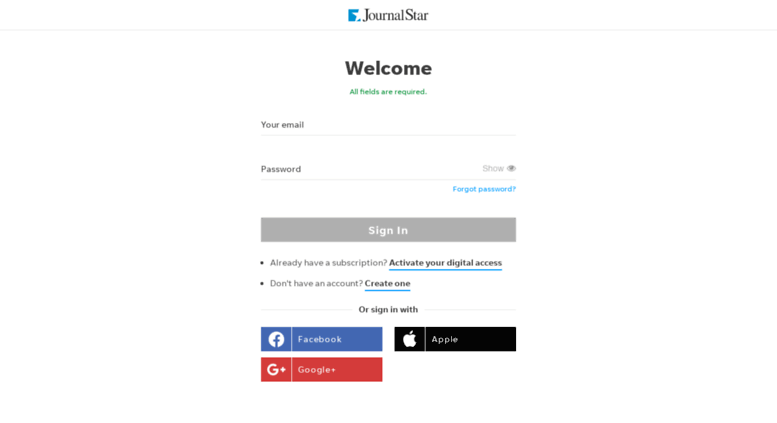This image appears to be a screenshot of a website log-in screen, characterized by its minimalistic design set against a white background. Centered at the top, the screen prominently features the text "Journal Star" in black font, accompanied by a small blue rectangle on its right side, which contains half of a white star. Below "Journal Star," the large, bold black text "Welcome" greets the user, followed by smaller green text stating "All fields are required."

The log-in interface is straightforward with two input fields: the first labeled "Your email" and the second "Password." The password field includes an additional feature on the right side—a "Show" option with an eye icon to reveal the password while typing. Beneath this, a blue link labeled "Forgot password" offers a way to recover lost login credentials.

A gray, rectangular button displaying "Sign in" in white font provides the means to initiate the login process. Below this, two bullet points offer further actions: the first one prompts existing subscribers to "Activate your digital access," with this phrase emphasized in bold, underlined black text with a blue underline. The second bullet point directs new users to "Create one," similarly styled in bold, underlined black text.

At the bottom, the screen offers alternative log-in methods under the heading "Or sign in with." Three buttons are available: a blue "Facebook" button with the Facebook logo on the top left, a black "Apple" button with the Apple logo on the right, and a red "Google Plus" button with the "G+" logo situated below the Facebook button.